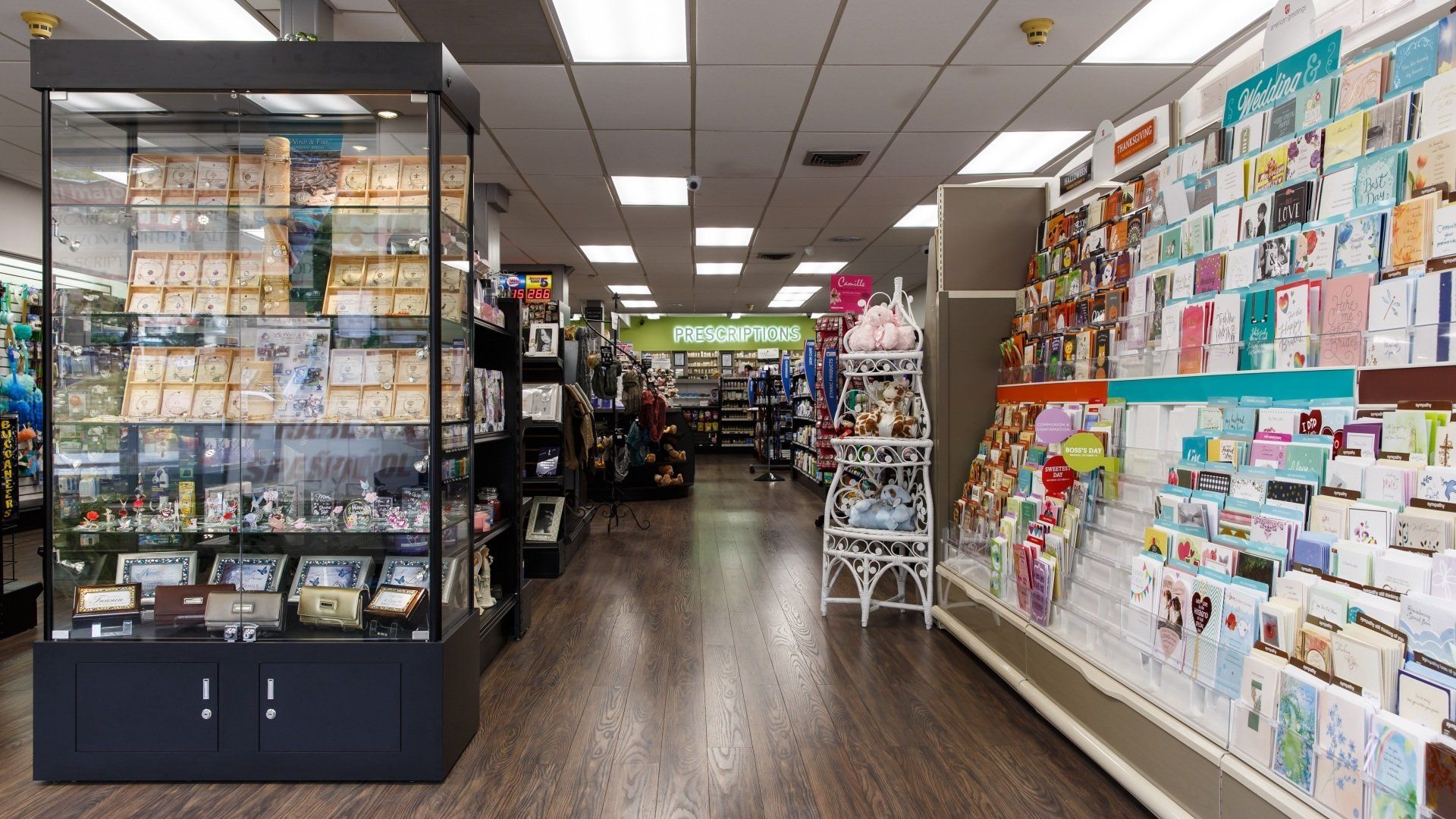The image depicts the interior of a store, potentially a pharmacy, illuminated by white lights set within a grey-tiled ceiling. The flooring is composed of wooden boards. On the extreme right side of the image, there is an assortment of gift cards in various colors ranging from red to pink, blue, and white. Towards the back of the store, there are shelves that appear to hold prescription medications, affirming the likelihood that this is a pharmacy. The left side features a large display case showcasing framed items, dolls, and figurines. Additionally, there are pictures adorning the walls. In the background, a person can be seen engaging in a conversation, adding a touch of liveliness to the scene.